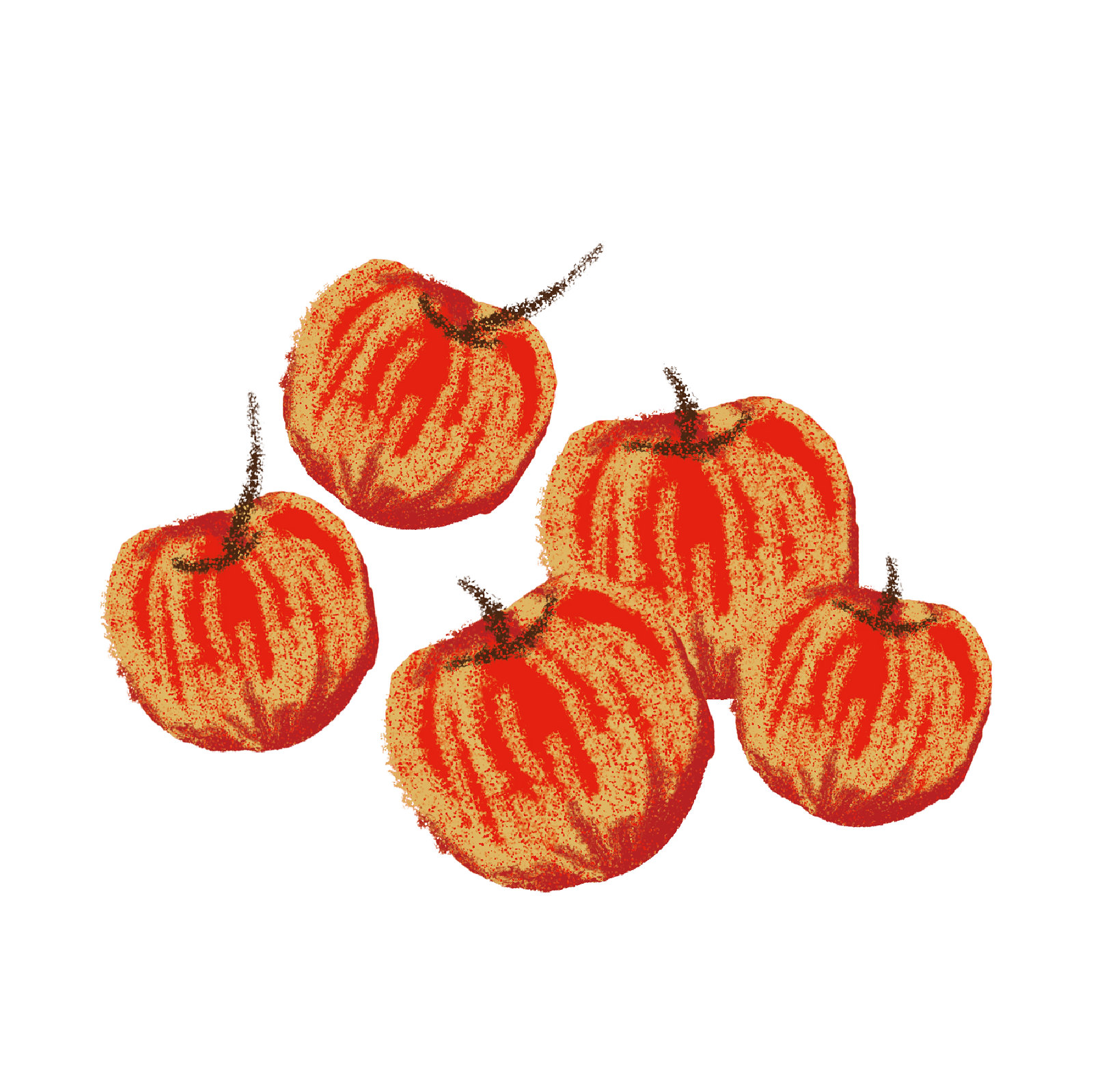This drawing features a hand-drawn depiction of five apples, each displaying a unique yet similar appearance, primarily created with crayon. The apples are vibrant red, resembling shades of crimson or scarlet, and transition to darker hues like burgundy or maroon near their bases. Their surfaces are adorned with vertical, slightly curved yellowish-tan streaks meant to depict texture or light reflection, somewhat reminiscent of peach fuzz. Each apple has a small, downward-curved black or brown indent at the top where the long, curved stems are attached. The apples vary slightly in size with one being particularly small, two medium, and two larger, all set against a stark white background that accentuates their bright colors. The drawing has no visible outlines for the apples, giving them a melded look with their surroundings.